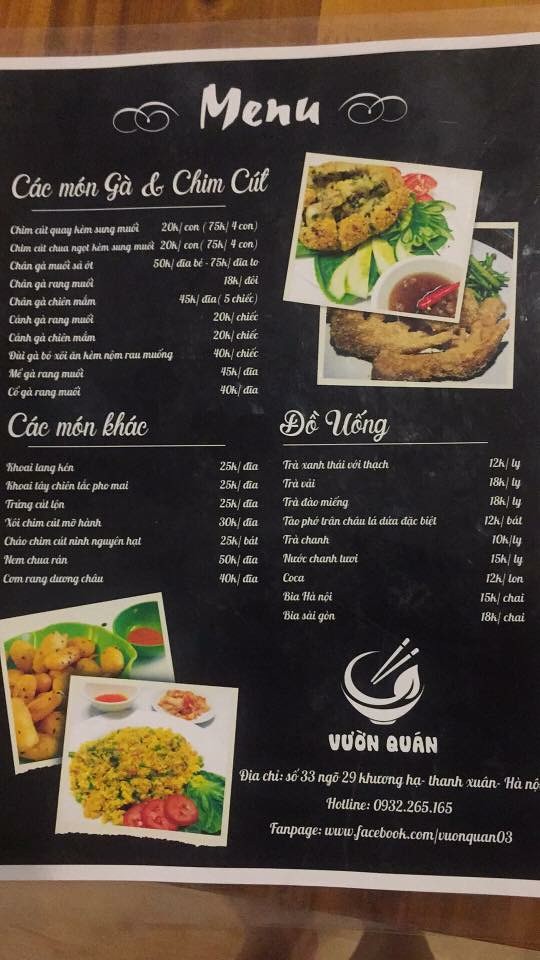The image appears to showcase a detailed, laminated menu placed on a wooden table. Along the bottom edge of the image, a portion of a person's leg and some of the brownish floor are visible, adding a touch of realism to the scene. The menu itself is bordered in white, and the main background is black with white text, which seems to describe Vietnamese dishes.

The menu is divided into three distinct sections: two on the left side and one on the bottom right. Above the bottom right section, there are two pictures, likely of some bread garnished with greens, possibly dumplings, and a sauce on the side. In the bottom left corner, there are additional images: one depicting a dish that appears to be rice with tomatoes, leaves, and some sauce, and the other of a dish that includes potatoes. The laminated paper of the menu extends about half an inch beyond its edges, adding a shiny finish. This meticulous arrangement and detail bring out the vividness and inviting nature of the menu, suggesting a rich and appetizing culinary experience.